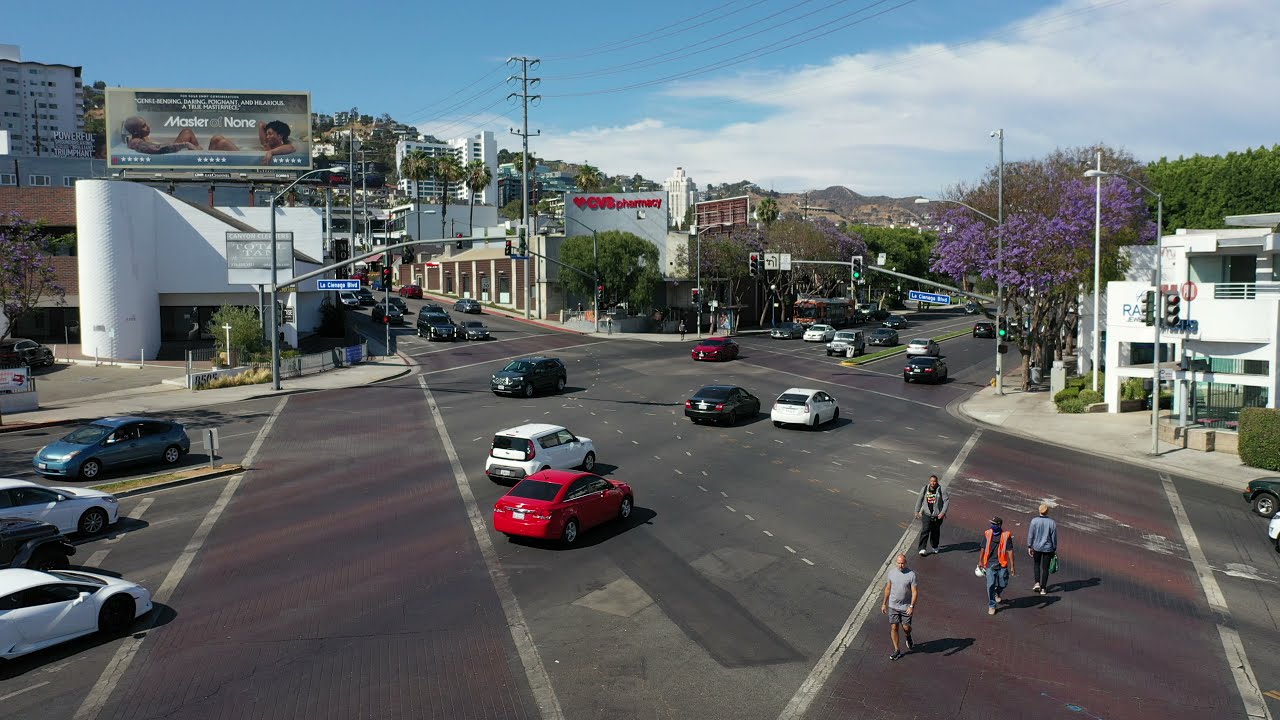The photograph captures a bustling four-way intersection where streets slightly diagonal to each other meet. In the foreground, several cars are driving in various directions, adhering to the green street light, while others wait to turn. The roads are relatively wide, accommodating two to three lanes of traffic each way.

Pedestrians navigate the crosswalk, including a city worker in an orange safety vest and a man leading the group in a gray t-shirt and shorts. On the right corner stands a CVS pharmacy, its white structure adorned with the iconic red CVS Pharmacy signage. Adjacent, a white commercial building sits at the base of a hill road.

Above the scene, telephone poles stretch across the sky, their wires threading through a backdrop of blue sky and white clouds. A prominent billboard on a nearby building advertises what appears to be a movie, featuring two people in a bathtub and the title "Master of None." In the distance, towering skyscrapers and residential buildings rise against the horizon, with more homes scattered on the hillsides, evoking the ambiance of a place like the Hollywood Hills. Punctuating the distant landscape are tall mountains, completing the vivid urban tableau.